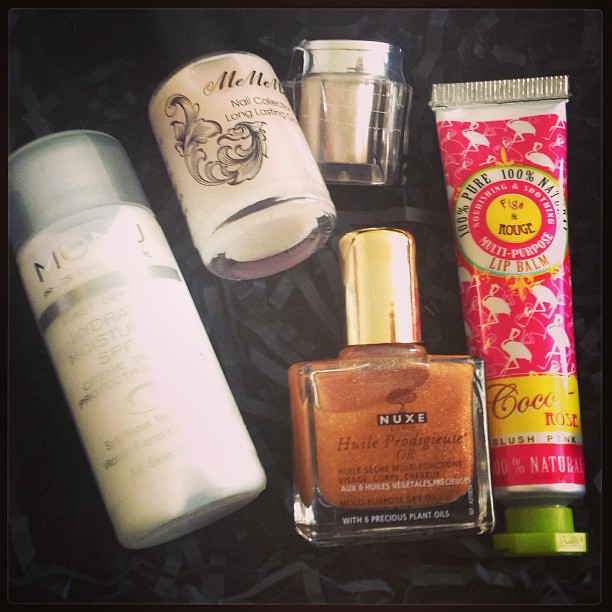The photograph depicts a curated arrangement of beauty products displayed on a bed of black shredded paper, resembling the type used in gift bags. From left to right, the items include:

1. A hydrating moisturizing SPF skin cream in an off-white bottle.
2. A slightly shorter glass bottle of long-lasting nail polish, likely with an off-white or pinkish hue.
3. A smaller glass container, possibly another variant of nail polish.
4. A larger bottle of reddish-orange nail polish.
5. A distinctive pink tube of 100% pure and natural multi-purpose lip balm, labeled "figs and rouge," adorned with flamingo outlines and capped with a green lid.

The products show varied uses ranging from skin hydration to nail and lip care, indicating a comprehensive selection of beauty essentials.